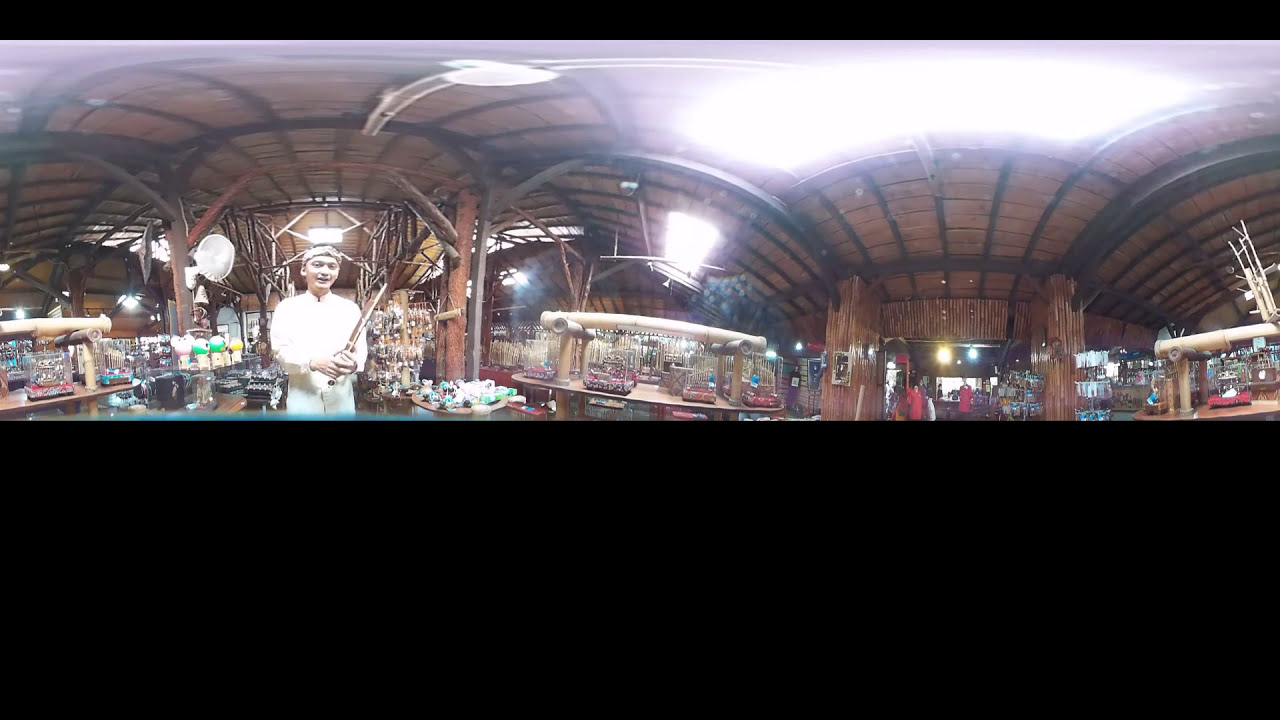The image depicts a 360-degree, panoramic view of the interior of an Asian-themed steakhouse restaurant. The room is brightly lit with fluorescent lights and has a ceiling made of black-framed, grid-style steel beams. The walls are wooden brown, complementing the warm ambiance of the space. At the center of the scene, a man dressed in a white chef’s uniform and a headband stands prominently, holding a sword or short knife. He faces the camera and is surrounded by multiple shelves filled with various small objects, toys, or figurines, adding to the decorative, cluttered charm of the restaurant. The tables are neatly arranged around the room, ready to accommodate diners. A fisheye lens effect distorts the image slightly but captures the essence of this lively, unique dining environment.